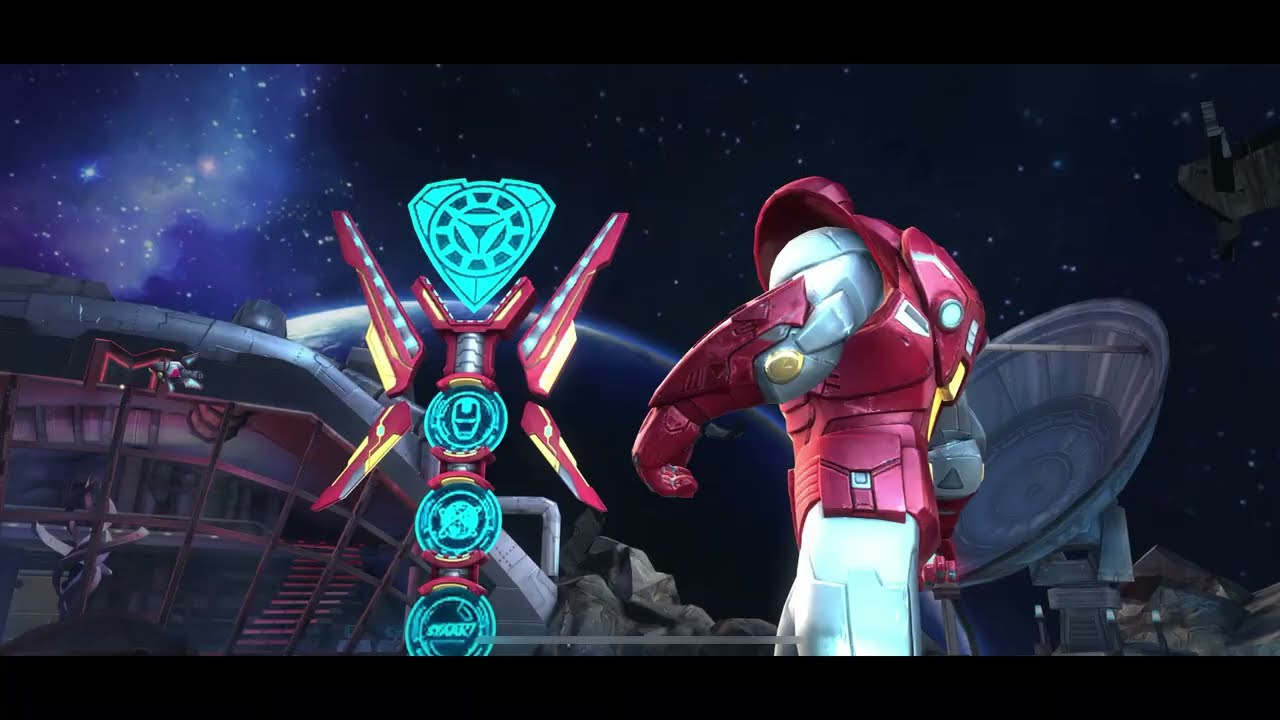The illustration appears to be a still shot from a video game or a poster based on one, rendered in a sophisticated, computerized art style. It depicts a humanoid figure, likely a robot or someone in an advanced suit of armor that resembles Iron Man, featuring a red metallic gauntlet and glove over a white or silver exoskeleton. The character is positioned slightly off-center to the right, from the shoulders to the waist clad in red armored plating. 

To the left of this figure, there is a futuristic pillar or totem-like structure, adorned with blue logos and red and yellow accents. This pillar includes three circles and an upside-down triangle in blue, and one logo notably resembles a blue Iron Man face. 

In the background, a modern-looking glass building and a metal satellite dish are visible. Above and beyond, a cosmic scene unfolds with a bright cluster of stars illuminating the upper left corner, transitioning to a darker sky with scattered stars on the right, indicating a nighttime setting in outer space. The entire composition is framed by thin black headers and footers, adding a cinematic feel to the artwork.